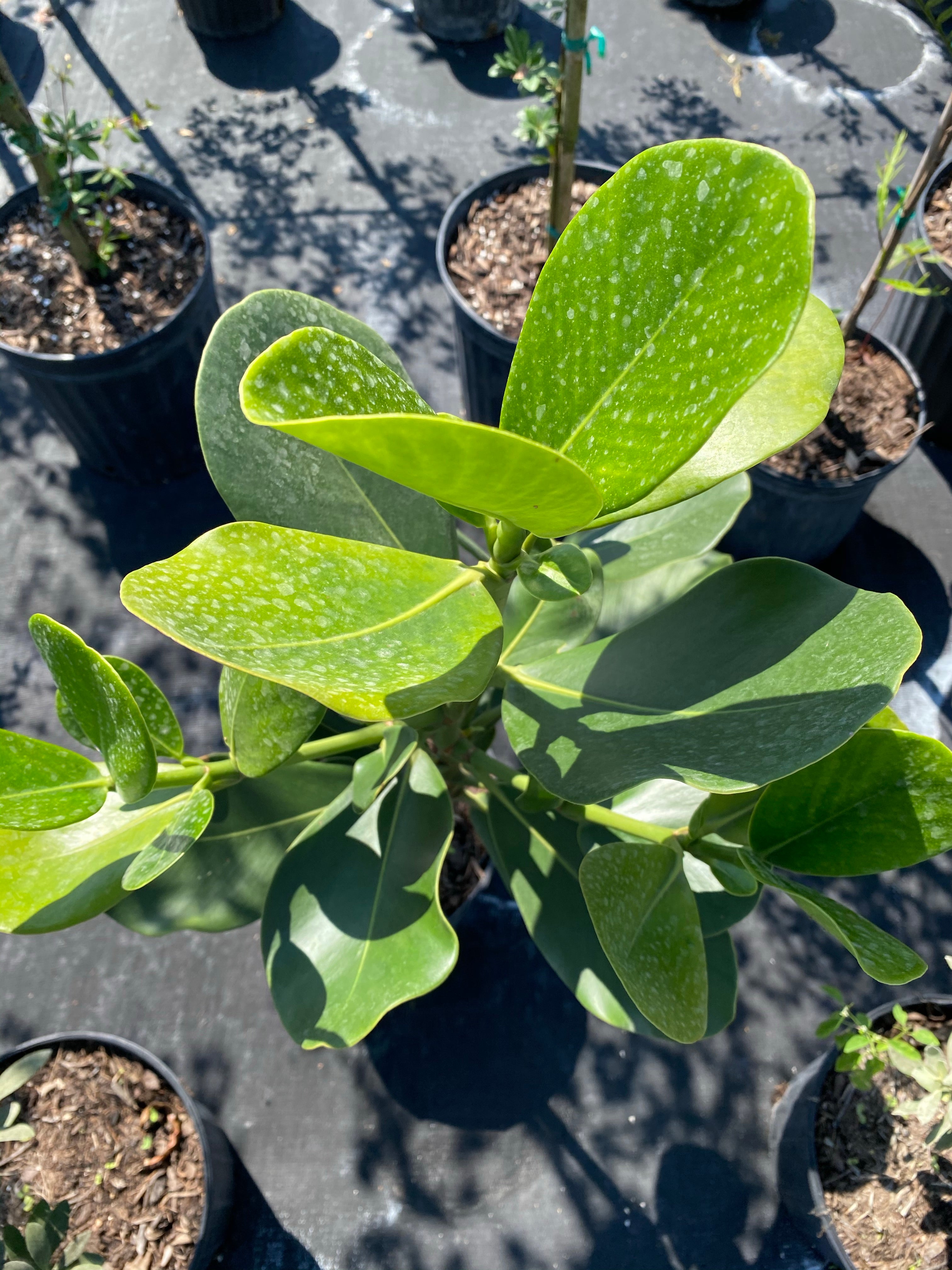This image is a close-up photograph taken from above, featuring a mature rubber tree plant in a black plastic pot. The plant's large, oval-shaped green leaves display white speckles, which could be water droplets or dirt. The leaves are thick and appear sturdy, oriented upwards with the top leaves noticeably brighter due to sunlight, casting shadows on the darker leaves below. Surrounding the main plant are several smaller potted plants with visible dirt and minimal greenery, indicating various stages of growth. The setting resembles a nursery, suggested by the arrangement of plants on an asphalt surface marked with chalk outlines from previously placed pots. Scattered stems in black pots and noticeable shadows due to the sunny weather enhance the scene's detail.